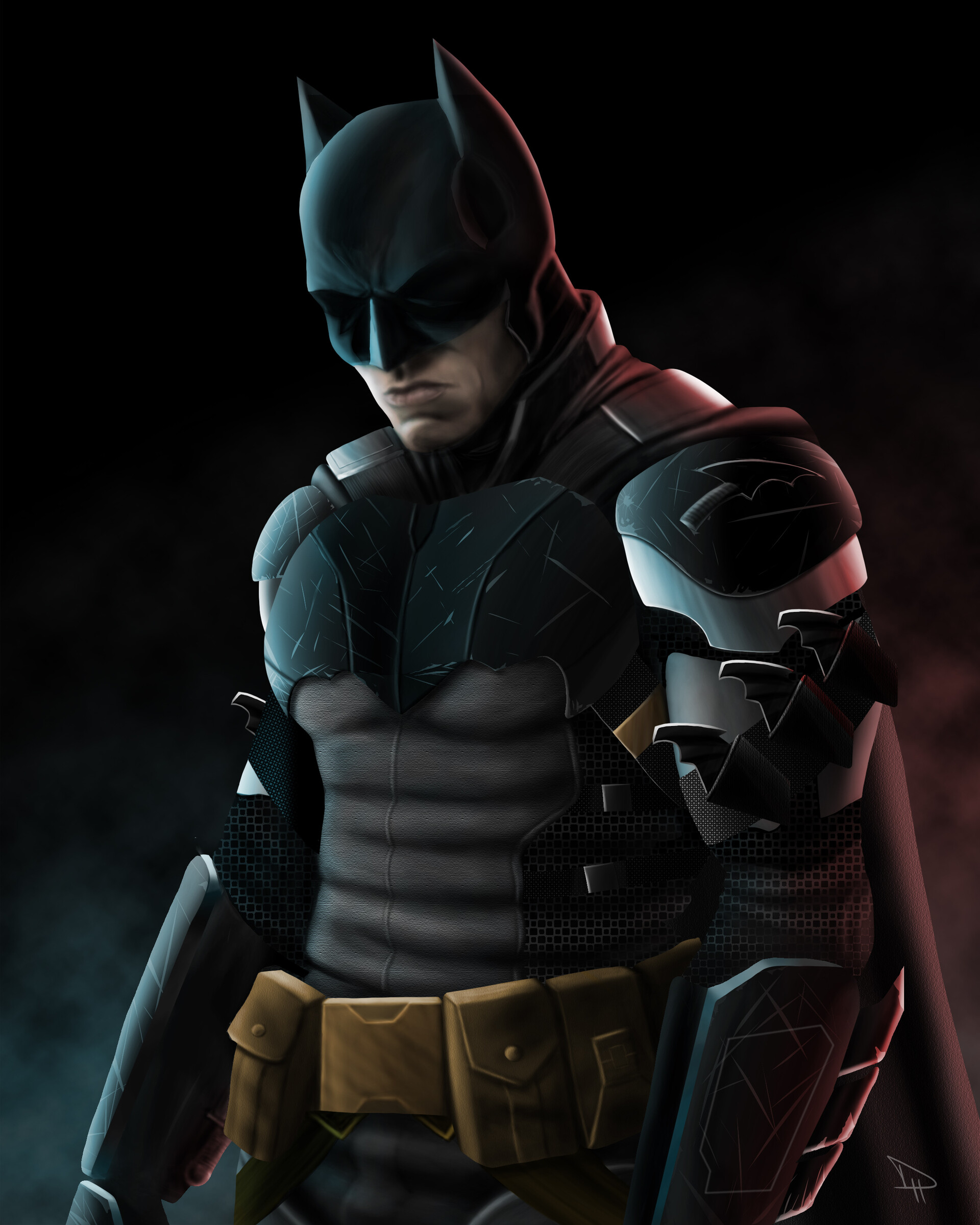This detailed digital rendering of Batman showcases a unique design that deviates from traditional depictions seen in movies or video games. Batman is centered in the image, with his torso prominent and his head slightly tilted downward. His iconic mask covers his eyes, extending up to his helmet-like headwear. The meticulously crafted suit includes notable elements such as metallic shoulder and bicep plates, with small batarangs attached, and a yellow-tan utility belt with multiple pockets.

The chest plate features a scratched bat symbol, subtly integrated into the armor. His cape, distinguished by metal bands over the shoulders, adds to the futuristic aesthetic. Batman is illuminated from the right side with warm red light, contrasting with the softer light on the left side. The background is predominantly black, enhancing the dramatic lighting and the ominous presence of the superhero. In the bottom right corner, there’s a small marking, likely a signature or logo of the artist. This piece, resembling concept art or a digital painting, emphasizes the modern and tactical approach to Batman's design.